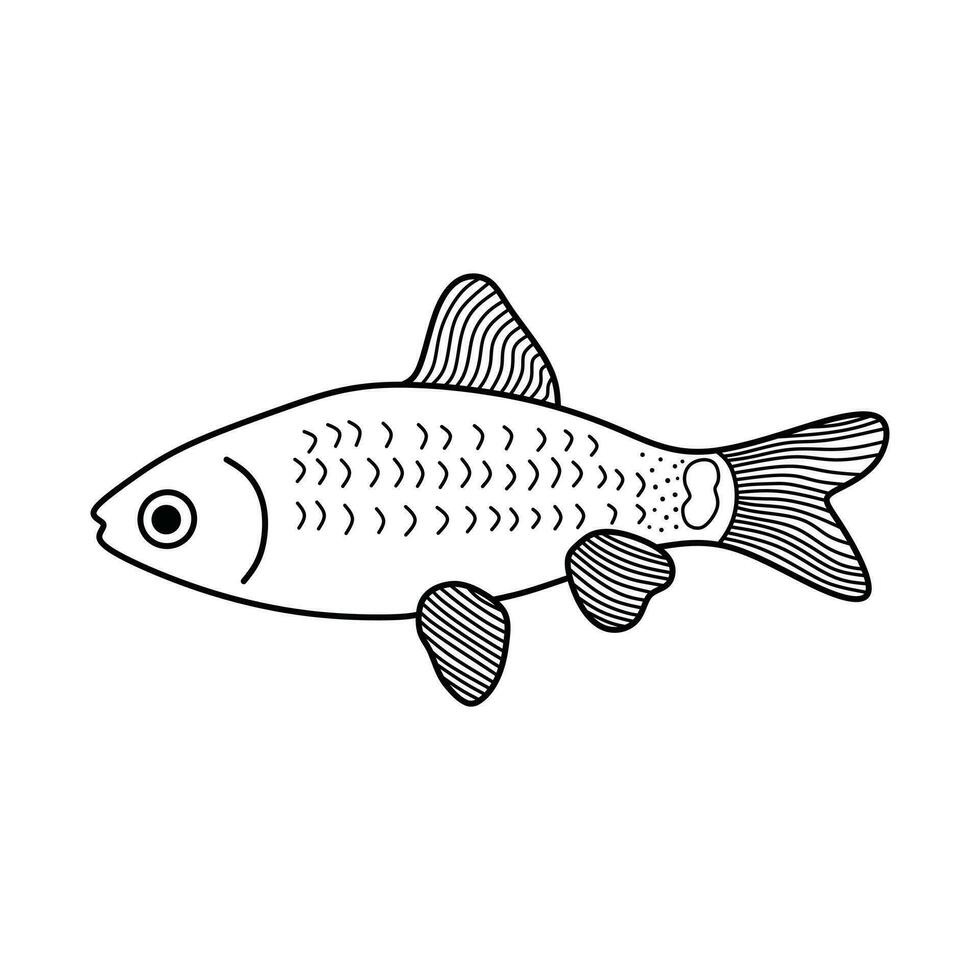This is an extremely simple, black and white line drawing of a fish, reminiscent of a basic illustration one might find in a children's coloring book. The fish is depicted swimming from left to right, with a round black eye encircled by a thin outline. Behind the eye, a single curved line signifies the gills, starting from the top and curving downwards. 

The fish has three fins: one dorsal fin on the top and two pectoral fins on the bottom. Each fin, along with the tail, is detailed with wavy or vertical lines to indicate texture. The body of the fish is adorned with small, gently curved semicircles to represent scales, and speckling near the tail end adds extra detail. The overall shape of the fish resembles a trout, with clearly defined, simple patterns and textures that make it easy to color and bring to life.